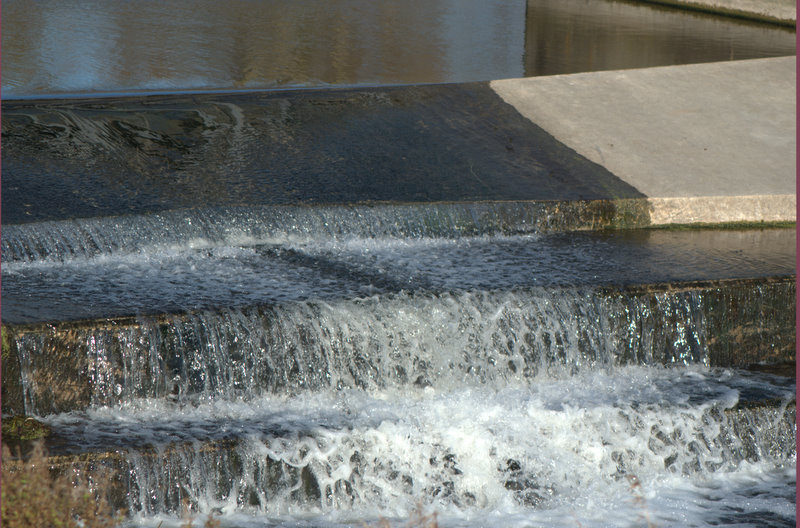This photograph captures an outdoor scene featuring a stepped water display, possibly part of a water monument or reservoir, located in what appears to be a park. The central focus is on three gray cement or stone steps, with water cascading down them, creating a miniature waterfall. The wet sections contrast sharply with the dry portions, highlighting the intended path of the water flow. Above the steps, a pool of water feeds the continuous stream, which generates a splashy white froth as it descends. The close-up view accentuates the dynamic motion of the water against the stark, plain background of the concrete or stone material. Reflections on the water surface confirm the outdoor setting, emphasizing the natural integration of this water feature within its surroundings.